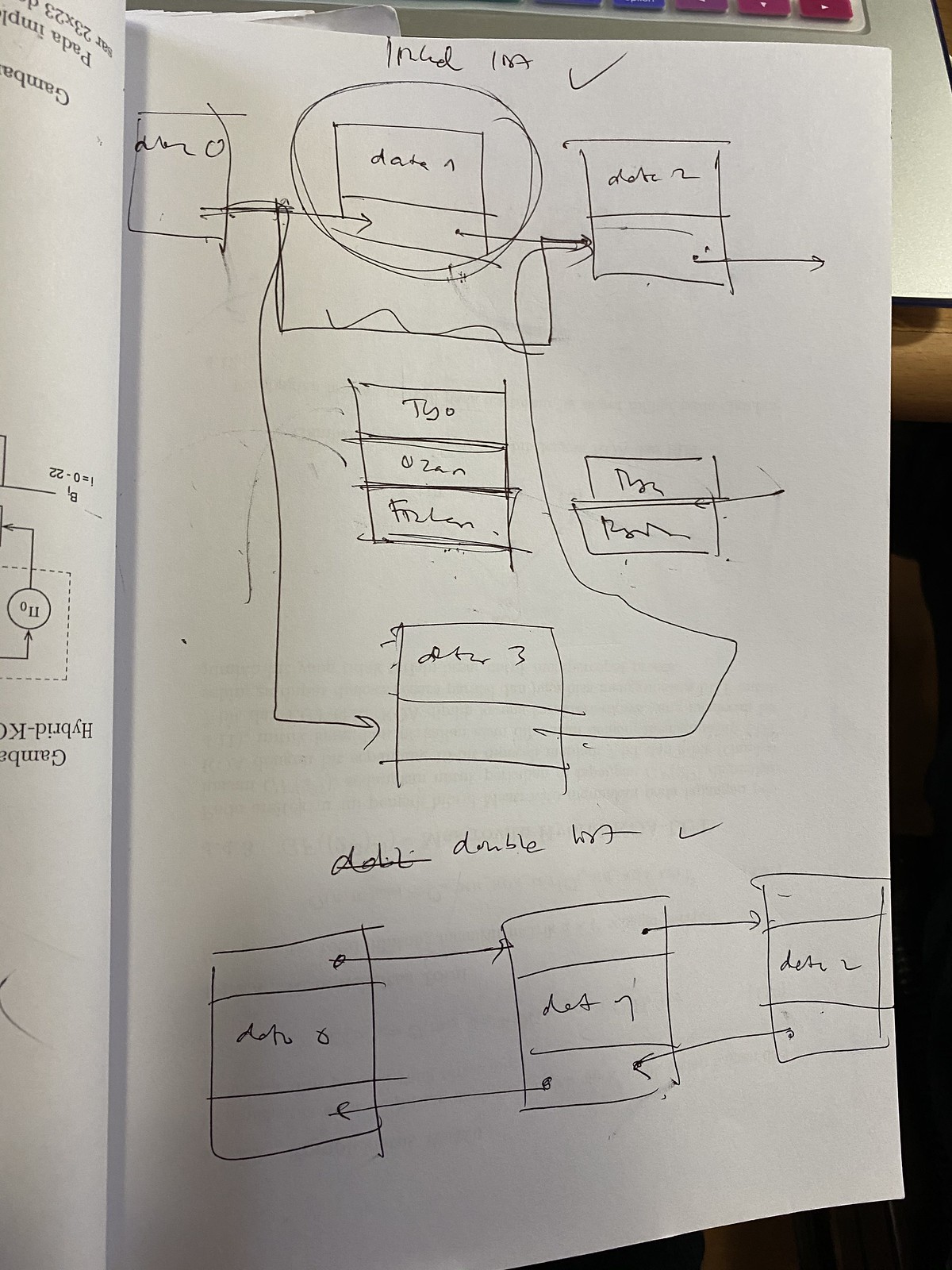A blank page from a workbook lies on a brown desk, partially resting against the keyboard of a laptop. The page is intended for note-taking, as suggested by the printed text on the adjacent page. A detailed and complex diagram spans the entire page. 

At the top of the diagram is a central circle containing a rectangle divided into two parts. Flanking this circle are two additional rectangles, each also divided into two parts. Arrows emanate from these rectangular sections, directing towards and away from the central circle, creating a loop. These arrows are interconnected by lines.

Below this loop, a singular, larger rectangle divided into three parts is connected by multiple lines to the upper sections. Directly beneath, there is another rectangle split into two sections, also linked to the diagram above by connecting lines.

Just below this lower rectangle, a phrase or sentence is written in what appears to be very messy cursive, which renders it nearly illegible. 

Further down the page, three more rectangles, each divided into three parts, are connected by arrows, continuing the complex network of shapes and connections. 

Overall, the diagram is intricate and detailed, illustrating a concept that appears to be heavily dependent on the visual flow created by the shapes and arrows.